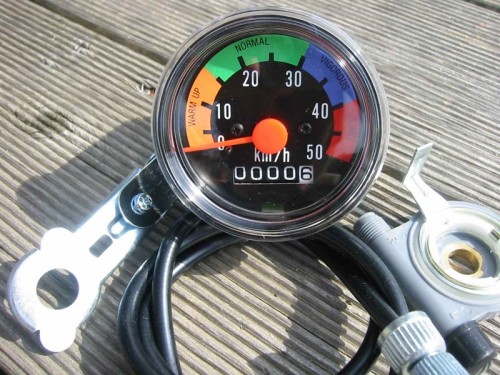The image depicts a gauge, possibly a speedometer, placed on what seems to be a picnic table or a corrugated flat box. The gauge is equipped with various nozzles which might connect to a device, likely a vehicle. The central feature is a black dial with an orange needle, marked with speed measurements in kilometers per hour, ranging from 0 to 50.

The dial is segmented into four color-coded zones with corresponding labels. The first segment, from 0 to 15 km/h, is marked in orange and labeled "Warm Up". The next segment, from 15 to 30 km/h, is green and labeled "Normal". The third segment, from 30 to 40 km/h, is labeled "Vigorous" and is colored yellow. The final segment, from 40 to 50 km/h, is red, but a glare on the image obscures the label in this section.

The gauge, which indicates that it has only traveled six kilometers, appears to be detached from its original vehicle or device. The complete odometer reading suggests it can go up to 99,999 kilometers.